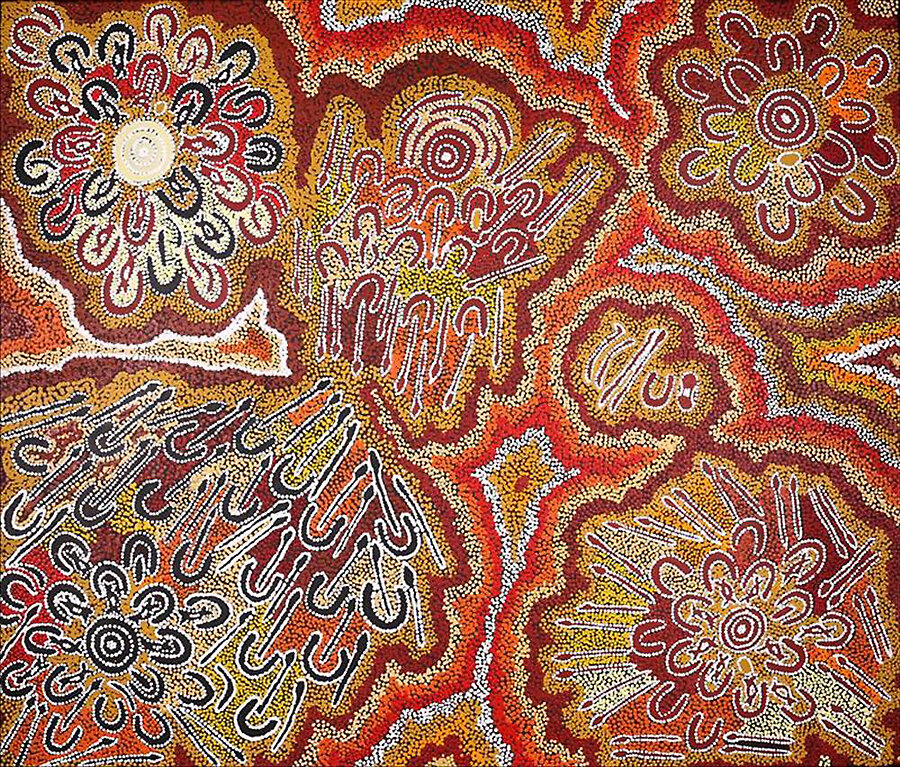The image is an intricate and colorful artwork that intricately blends various design elements. It features a kaleidoscopic scene reminiscent of a mandala, but it isn't perfectly symmetrical. This tapestry-like piece, possibly resembling an African textile or Aboriginal artwork, is created with what looks like individual beads or dots of paint glued together. The color palette includes earth tones such as burnt orange, mustard yellow, rusty red, light yellow, white, black, and some cream-colored accents. These vibrant hues form numerous distinct scenes with circular centers surrounded by horseshoe or U-shaped patterns, suggestive of floral designs. Upon closer inspection, there are stylized representations of spears, shields, boomerangs, and other shapes like hourglasses and squiggly lines, contributing to the sense of an abstract battle or symbolic display. The meticulous arrangement of shapes and colors gives the overall appearance of being a finely detailed psychedelic rug.